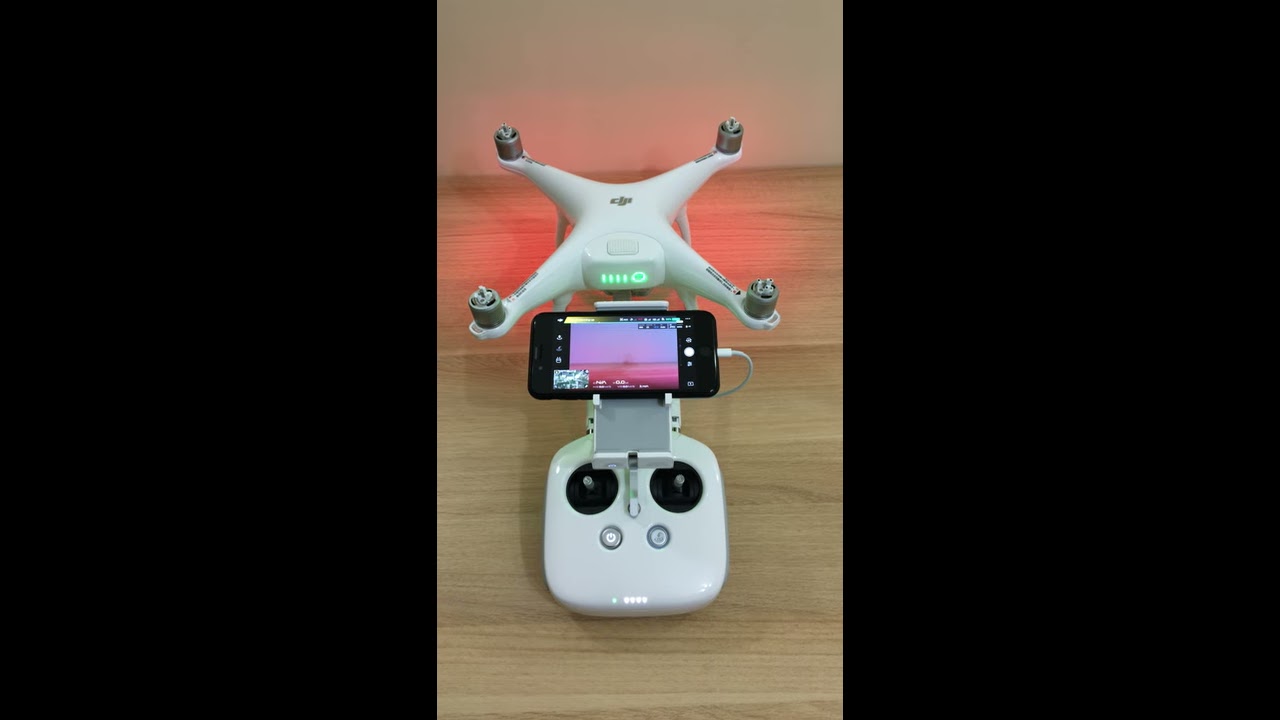This photograph depicts a detailed indoor scene centered on a drone, which is positioned on a brown wooden table. The image is formatted as a triptych, with the focal point being the clearly captured middle panel, while the left and right panels are out of focus. The drone itself is dark gray with light gray accents and features four propellers arranged in an X shape. Attached to the drone is a black smartphone, connected by a USB cable running to the base of the drone. This base, or controller, is off-white, with two prominent black circular controls on either side and two smaller gray buttons. The smartphone's screen is illuminated, suggesting it is powered on and recording. Further adding to the composition, a red light is visible in the background, casting a reflection on the table and subtly illuminating the scene. No readable text is present in the image. The setting includes a glimpse of a white wall in the upper part of the image, giving a contextual hint of the indoor environment.